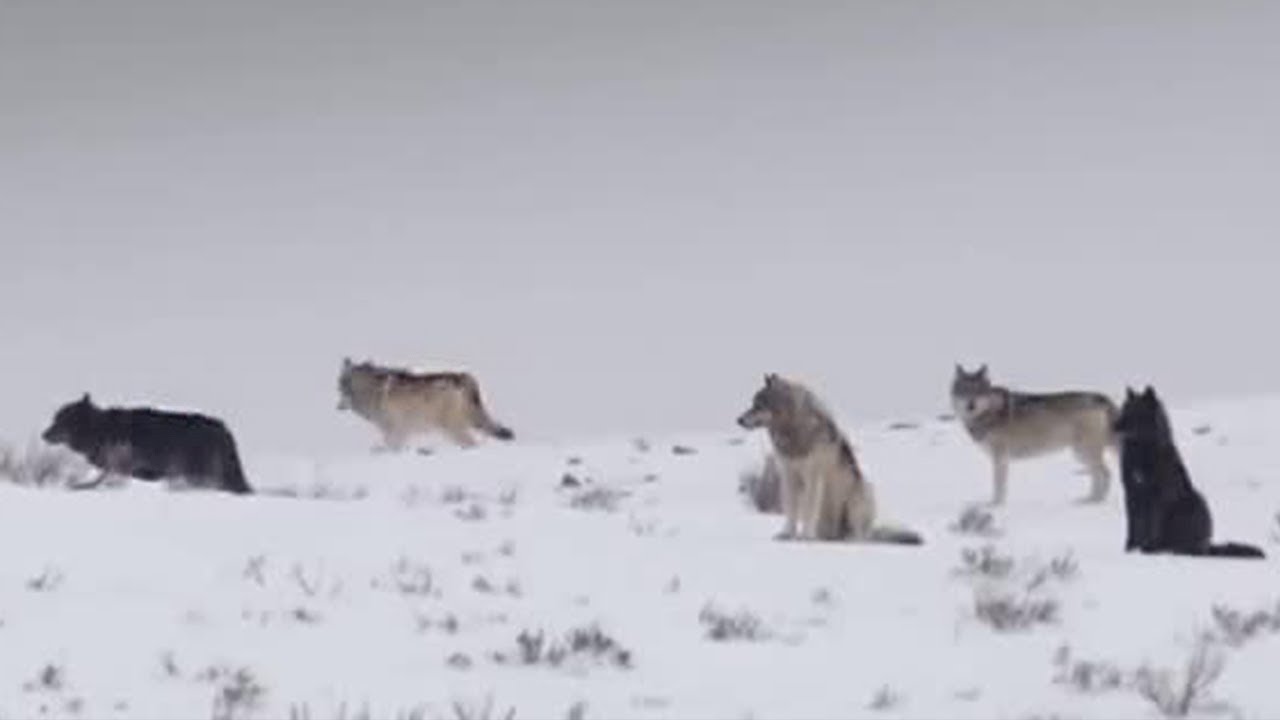In this image, we observe a pack of five wolves situated in a snowy, open field. The scene includes two black wolves and three gray wolves, all distinctively arranged in the winter landscape. On the left side of the image, a black wolf and a gray wolf are both walking towards the left. Centered in the image is another gray wolf, sitting down, while a fourth gray wolf stands beside it, looking directly at the camera. The last wolf, also black, is seated towards the background. The setting is bleak and wintry, with a gray, overcast sky and snow-covered ground interspersed with sparse patches of sticks and twigs. The image has a blurry, foggy appearance, giving it an aged look. The wolves appear alert and attentive in this cold, snowy environment.